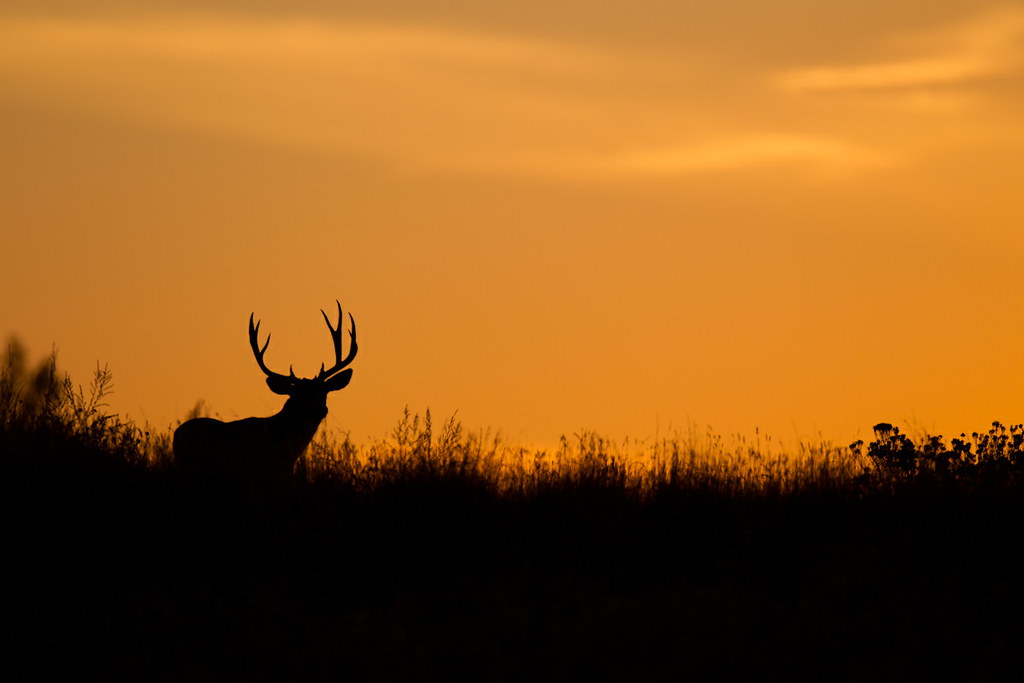The photograph captures a striking silhouette of a well-antlered stag positioned on the left side of the image, set against the mesmerizing backdrop of a sunset over a prairie or grassland in what could be the western United States. The stag's impressive antlers, featuring at least nine or a dozen points, dominate the scene as they rise prominently from its head. The animal is partly obscured by tall grasses, which, along with a few bare trees and shrubs, form a dark, uniform lower portion of the image. These elements stand out starkly against the vivid, almost uniform orange sky, variably shaded by clouds that play with the light's opacity. The sky, transitioning from a rich orangish-brownish-yellow near the horizon to slightly darker hues, envelops the entire scene in a warm, glowing light, emphasizing the striking contrast between the silhouetted landscape and the brilliant sunset. This ethereal tableau not only highlights the majestic deer but also beautifully captures the serene expanse of the grasslands at dusk.